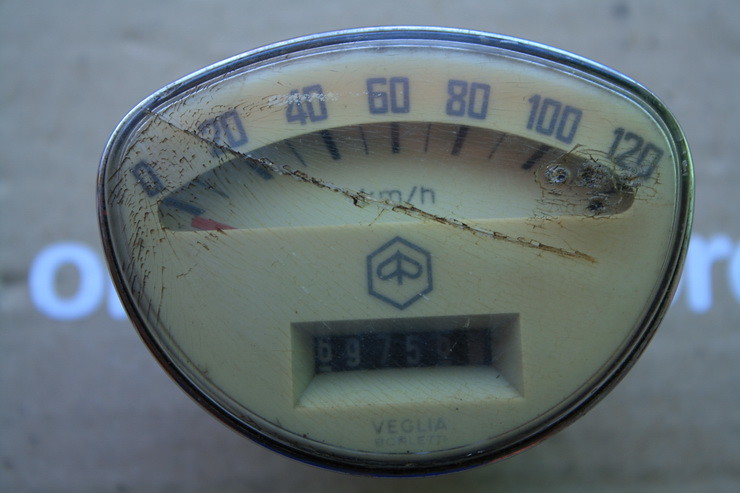A close-up photo captures an extremely vintage speedometer and odometer unit, detached and resting on a surface. The instrument, with an oblong shape, displays a speed range from 0 to 120 kilometers per hour using an analog dial. The tip of a red indicator rests on the left side of the gauge. The surface of the jewel glass is notably damaged, featuring cracks and stains that attest to its age. The odometer, located in the lower recessed portion, shows the numbers 6, 9, 7, 5, although the last two digits are obscured and unreadable. The brand "VEGLIA" is prominently displayed, with chrome edges framing the device. The background is out of focus, with indistinct letters, including an 'O' and an 'R', in light blue against a medium gray backdrop. The instrument itself has an off-white, almost cream-colored face, accentuating its vintage charm and wear.